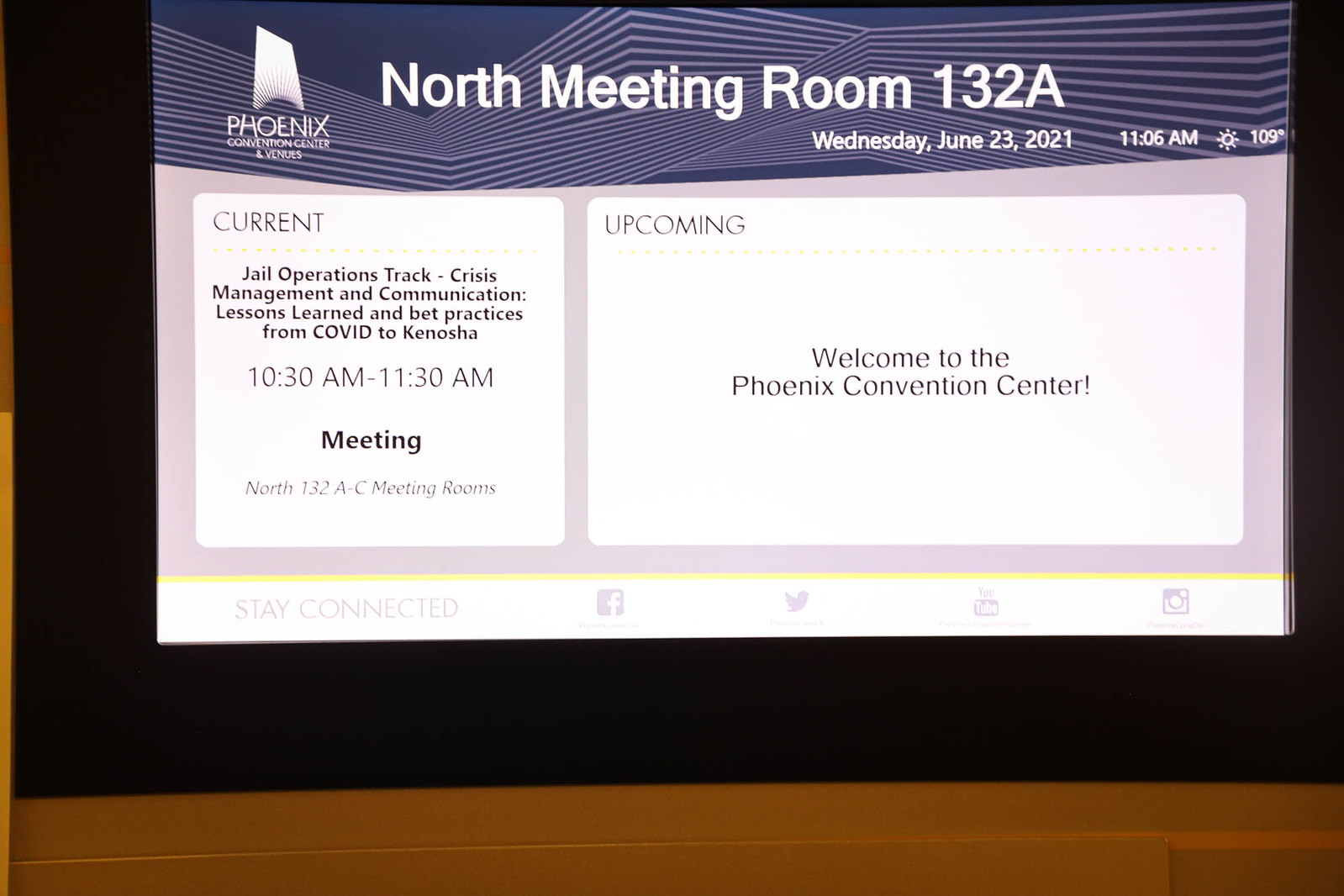The image appears to be a rectangular PowerPoint slide projected onto a wall, with a light brown border at the bottom. The slide's main background is black, and the content is framed within this black area. At the top, against a blue background with angular pinkish-purple lines, white sans-serif text reads "North Meeting Room 132A." To the left, a white symbol and text indicate "Phoenix Convention Center and Venues," featuring a logo depicting a building with sun rays. Below "North Meeting Room 132A," in smaller white text, it states "Wednesday, June 23rd, 2021, 11:06 a.m." along with a sun icon displaying "109°."

The slide is divided into two main sections with white backgrounds set within light purple borders. The left section, square-shaped, is titled "Current" in black text above a yellow dotted line. It details: "Jail Operations Track: Crisis Management and Communication Lessons Learned and Vet Practices from COVID to Kenosha, 10:30 a.m. to 11:30 a.m., Meeting, North 132A-C Meeting Rooms." The right section is labeled "Upcoming" above another yellow dotted line, followed by "Welcome to the Phoenix Convention Center" in the center. 

At the bottom of the slide is a yellow pinstripe line and a white footer. In light purple text, it reads "Stay Connected," accompanied by logos for Facebook, Twitter, YouTube, and Instagram.